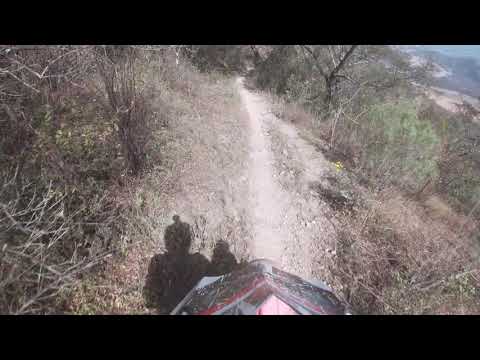In this vibrant color photograph, we observe the perspective of someone riding a motorcycle or dirt bike down a light brown, dry dirt trail set on the side of a fairly steep mountain. The multicolored cowl of the motorbike is prominently visible, bearing a mix of pink, blue, red, and gray hues, and appears scratched up. Just in front of it is a notable plastic arch. The rider, whose shadow is cast on the trail, is wearing a helmet, likely equipped with a mounted camera.

On the left side of the path, the terrain slopes upward, revealing a mix of gray vegetation, dirt, dead sticks, and sporadic green weeds. On the right, the slope descends sharply, dotted mostly with dead twigs and one notable green bush with a wealth of leaves. Further along the trail, a few sparse trees that look dormant for the winter stand stark against the backdrop. However, in the distance, some trees with green leaves can be seen lining the trail, adding a patch of vibrancy to the scene. The sky is clear blue, suggesting a sunny day, and in the upper right-hand corner, there appears to be a glimpse of a distant body of water. The overall impression is one of isolation, with no other riders visible, emphasizing the solitary nature of the journey.